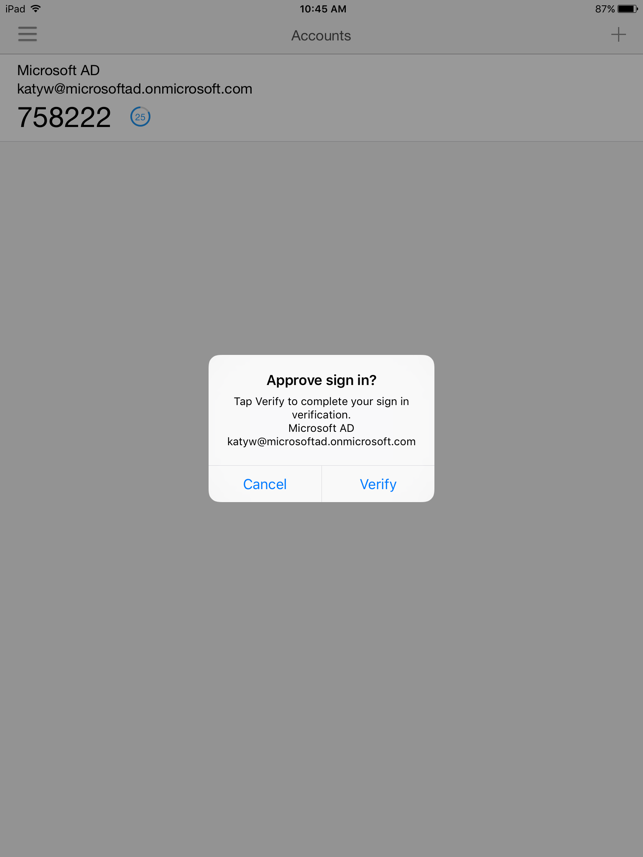The image displays a user interface pop-up from a Microsoft sign-in verification screen on an iPad. The pop-up box is a super light gray rectangle with a prominent black, bold header that reads "Approve." Below it, still in black and bold, is a question: "Sign in?" This is followed by a directive in standard font: "Tap verify to complete your sign-in verification." At the bottom in standard font, it mentions "Microsoft AD" and "KDW at Microsoft.com."

Within the pop-up, there are two blue buttons: one labeled "Cancel" and the other "Verify." The overall background of the screen is gray.

In the upper-left corner of the pop-up, black text reads "iPad," accompanied by black Wi-Fi signal bars. Centrally, it displays the time as "10:45 AM." On the right side, the battery percentage is shown as "87%" in black text.

Below the pop-up, there is additional information displayed on the screen:
- On the left-hand side, there are three horizontal gray lines next to the word "Accounts."
- Centrally aligned, it displays "Accounts."
- On the right side, there is a plus sign (+).

Further below, with a white background, the screen shows "Microsoft AD," followed by "KDW at Microsoft.com." Large, bold numbers "758222" are displayed prominently.

This detailed caption captures both the layout and the specific textual details of the screen, providing a comprehensive description of the visual elements.